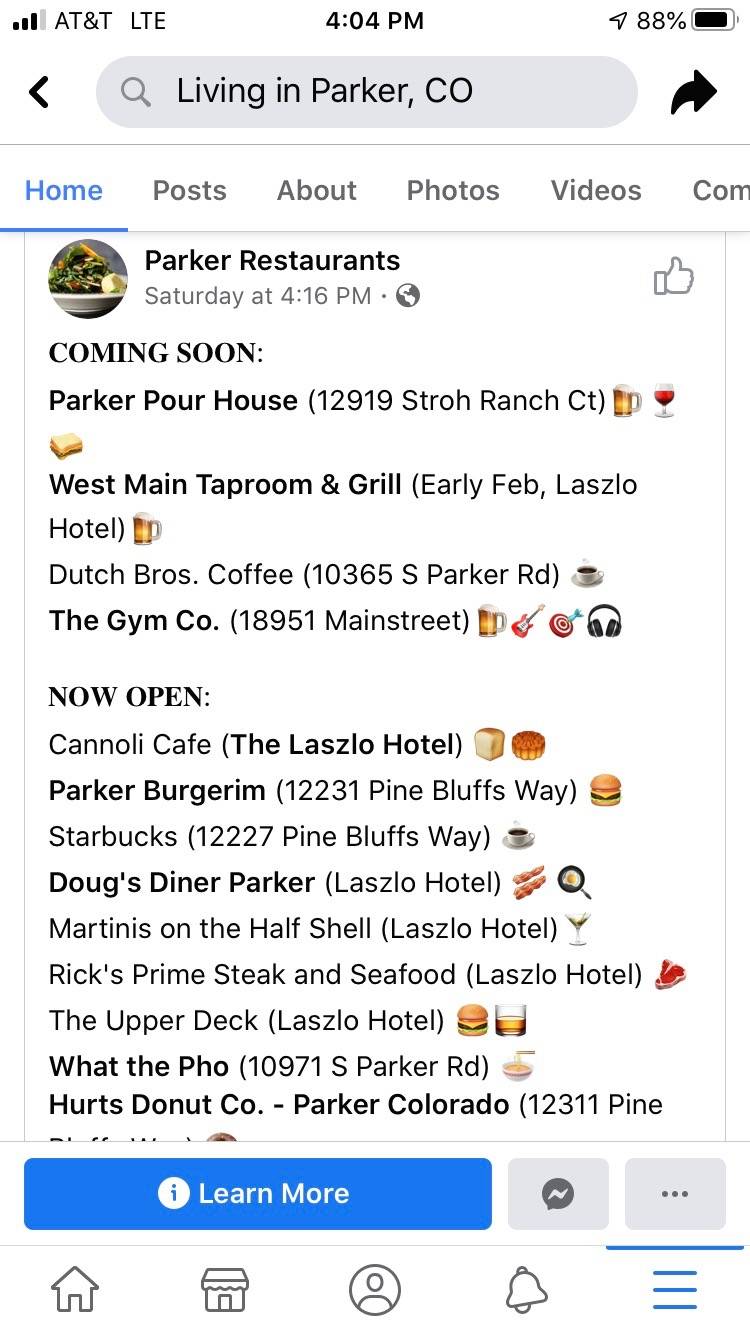Here is a cleaned-up and detailed caption for the image described:

---

The image displays a screenshot of an iPhone home screen. At the top left corner, the network signal bar indicates the device is connected to AT&T's LTE service. The time displayed at the center top of the screen is 4:04 PM. On the top right, the battery indicator shows an 88% charge. The main content of the screenshot is an open Facebook app. The search field at the top reads "living in Parker, CO." Below the search bar are various clickable tabs such as Home, Posts, About, Photos, Videos, and Parker Restaurants.

The timeline shows a post stating "Saturday at 4:16 PM," announcing "Coming Soon: Parker Paw House" at the address 12919 Straw Ranch, City. Mentioned locations include West Main Taproom and Grill, set to open in early February, and Lazy Hotel. Other businesses listed are Dutch Bros Coffee at 10365 S Parker Road, The Gym Co. located at 18951 Main Street, which is marked as "Now Open," and Cannoli Cafe. Parker Burger situated at 12231 Pine is also mentioned.

---

This refined caption provides a comprehensive description of the various elements visible in the screenshot, enhancing clarity and detail.